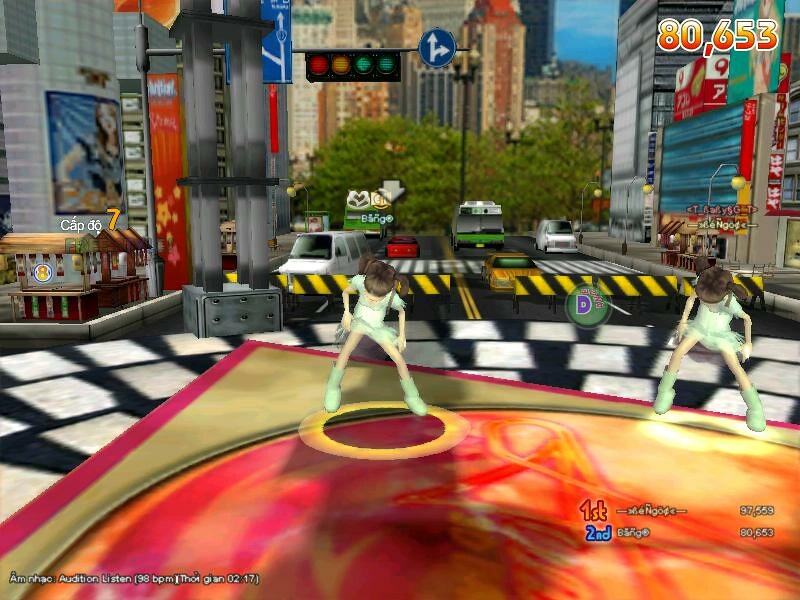In this vibrant and dynamic video game screenshot, two animated female characters stand confidently with their legs apart, ready for action. Both clad in matching green outfits with skirts and green boots, they are distinguishable by their hairstyles: one sports pigtails while the other has a ponytail. The scene is set within a vividly decorated ring, which is embedded with multicolored shades of yellow, pink, and orange. One of the characters is captured mid-jump, aiming to land in another colorful ring in the foreground. The backdrop features a bustling city block adorned with tall buildings, various vehicles in traffic, and lush trees. Architectural elements like a subway entrance and checkered black-and-white flooring add depth to the urban landscape. Additionally, some buildings are adorned with Asian writing, emphasizing the game's culturally rich setting.